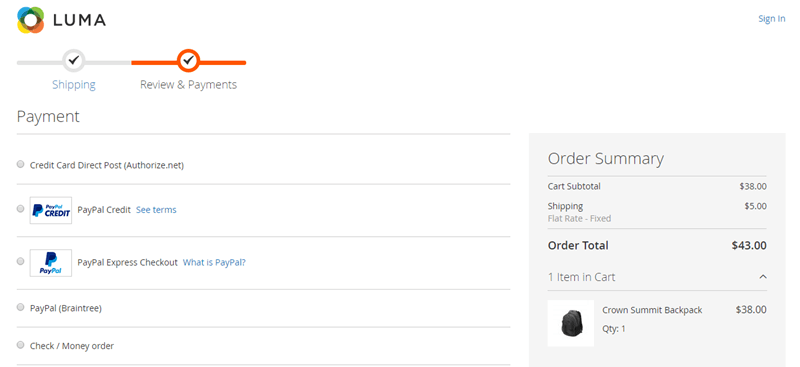This screenshot captures the payment page of the Luma website. In the top left corner, the word "Luma" is prominently displayed in black font, accompanied by the Luma logo. The logo features a white circle encased in multicolored bars that form a symmetric, star-like design with four rounded edges.

Beneath the Luma logo, there's a progress bar indicating the checkout steps. The "Shipping" section is grayed out and marked with a checkmark, signifying its completion. The "Payment" section of the progress bar is highlighted in orange, indicating that this is the current step the user is on. 

Below the progress bar, the payment options are listed: "Credit Card," "Direct Post," "PayPal Credit," and "PayPal Express Checkout." To the right of these options, the total amount for the order is displayed as $43.00.